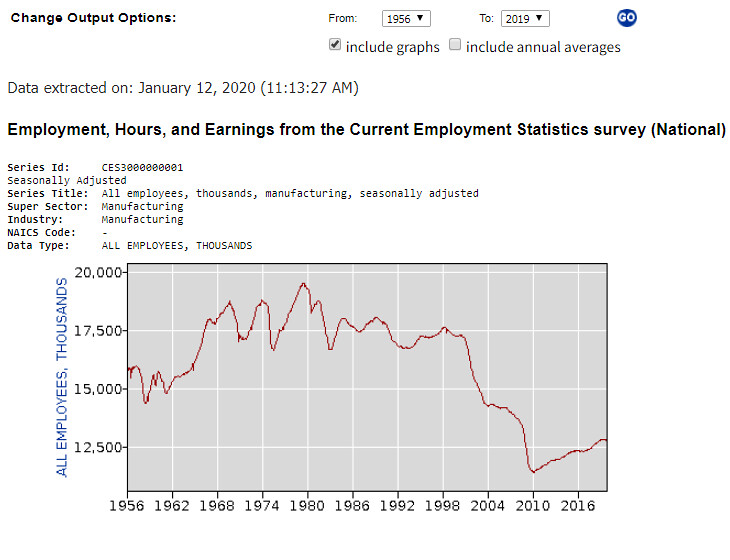This is a detailed caption describing a line graph illustrating employment hours and earnings based on data from the Current Employment Statistics Survey (National). The graph, set against a gray background, features a fluctuating red line charting the number of employees, measured in thousands from 12,500 to 20,000, across various years listed along the bottom: 1956, 1962, 1968, 1974, 1980, 1986, 1992, 1998, 2004, 2010, and 2016.

In the upper left-hand corner of the image, there is black text that reads "Change Output Options." To the right, it notes the data range from 1956 to 2019. Below this, it says "Include Graphs," with an adjacent check mark, and "Include Annual Averages," next to an empty check box. Further down, it specifies that the data was extracted on "January 12, 2020, 11:13:27 AM." Just above the graph, there's additional text that reads "Employment hours and earnings from the Current Employment Statistics Survey (National)."

This line graph provides a historical view of employment trends over more than five decades, with the y-axis indicating employee numbers in thousands and the x-axis charting the progression of years.